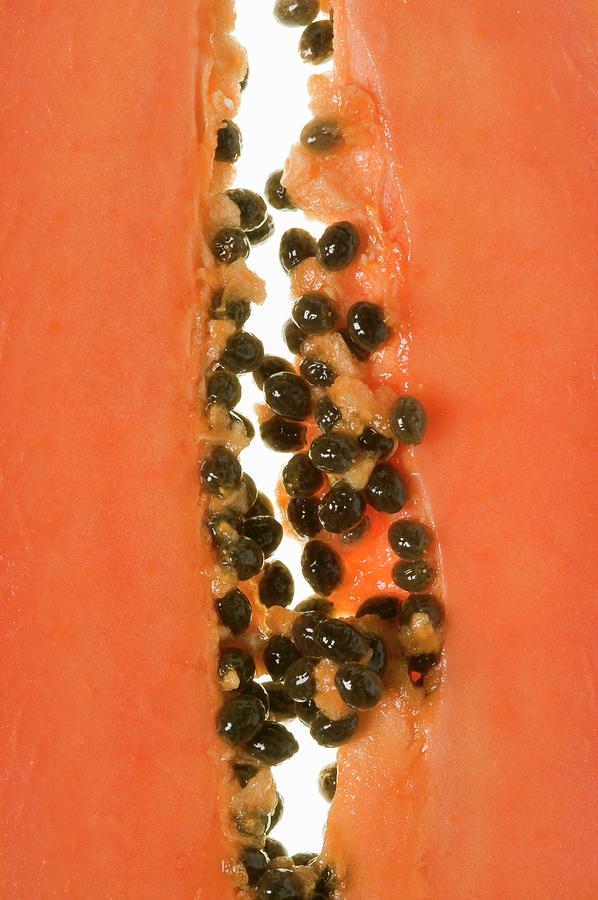The rectangular image depicts a vivid and unsettling scene. The edges of the rectangle are framed in a coral color, giving a vibrant yet eerie border. In the center lies an image resembling a severe, exposed wound with an oozy, jelly-like texture. The flesh-like area showcases a glossy, glistening quality, matching the coral hue but with a more intense shine. The wound is filled with what appear to be black, shiny spheres, akin to caviar or jelly beans made of licorice. Interspersed within these black spheres are small particles that resemble segments of an orange, adding contrasting colors and textures to the already intricate and disconcerting composition.